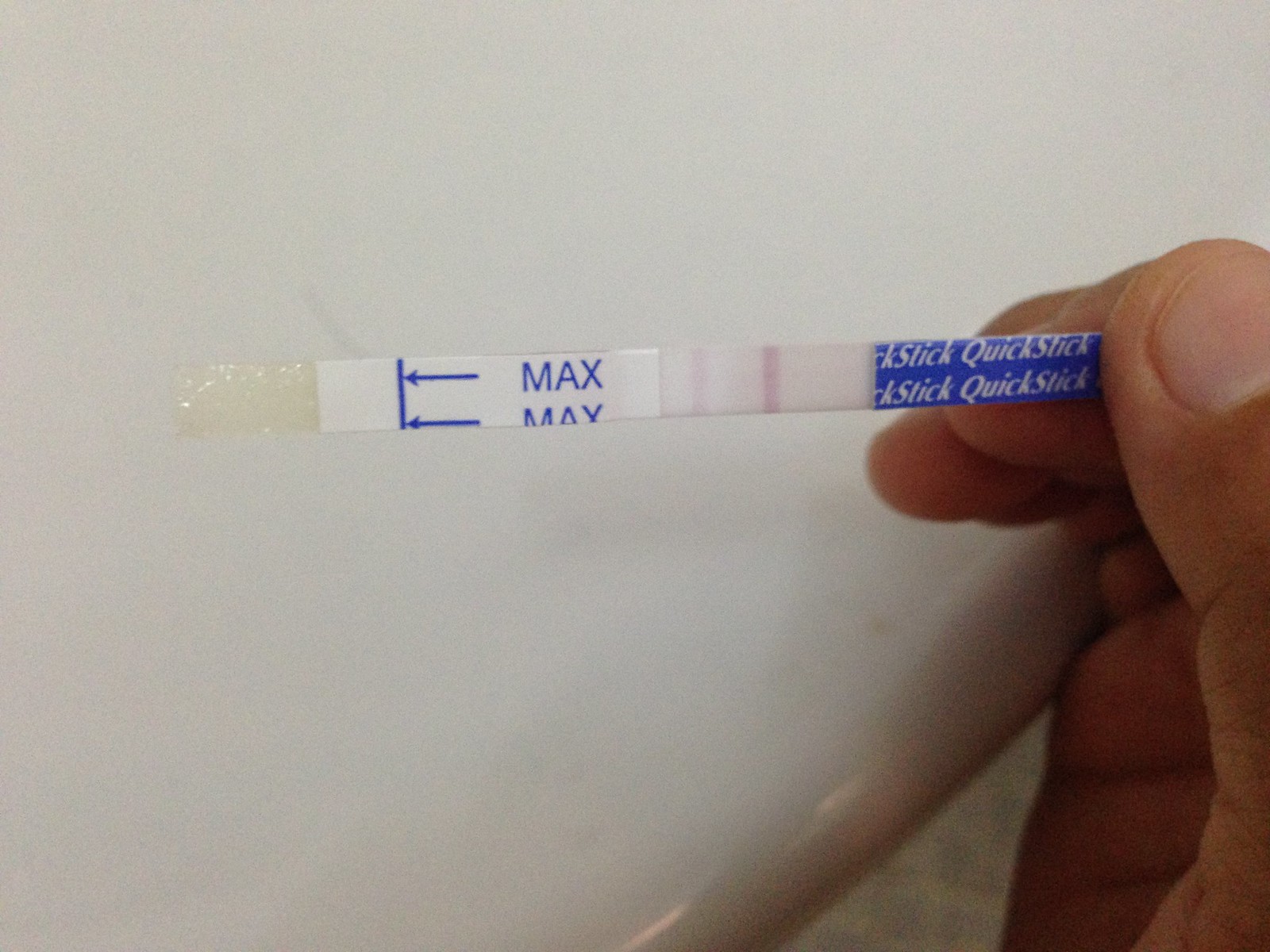In this photograph, the focus is on a white man's right hand, specifically the thumb and first two fingers, holding a thin test strip roughly three inches in length. The strip gradients from a liquid-like substance at its far left end to a white section that features the word "MAX" and an arrow pointing left. Approximately an inch to the right of the white section, the strip turns blue and is labeled with the text "quick stick" repeated twice. The precise purpose of this test strip is unclear from the image. The detailed elements and labels on the strip suggest a diagnostic or monitoring function.